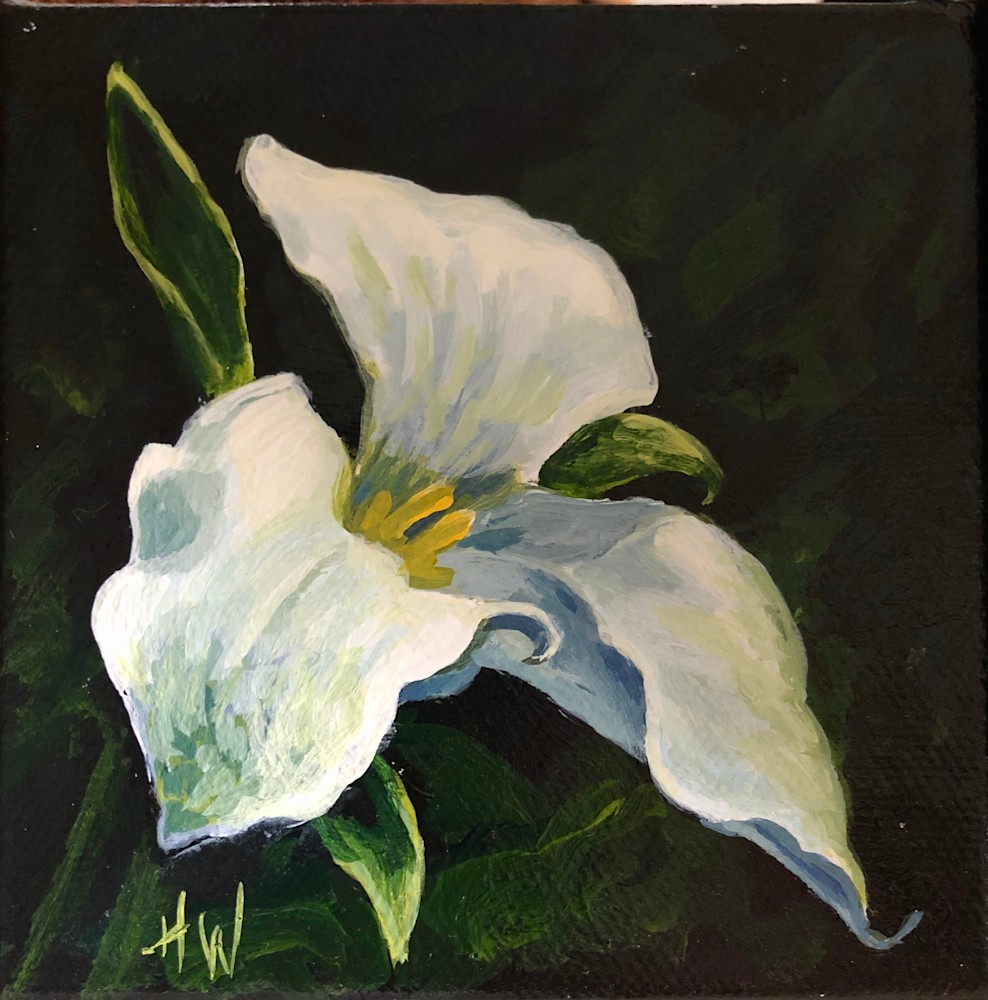This oil painting on canvas showcases a detailed white iris flower with three large, somewhat cone-shaped petals that point and drape downwards, giving them a furl-like appearance. Each petal is subtly highlighted with hints of green, contributing to their realistic texture. A vibrant yellow pistil, or stamina, is centrally located within the flower, adding a touch of contrast. The flower is framed by three green leaves, each delicately edged with light green or white. The richly textured background features dark shades of forest green interwoven with black, creating a deep and intricate backdrop. At the bottom left of the painting, the artist has signed their initials "HW" in a light green color, blending seamlessly with the overall color scheme. The meticulous brushwork captures both the beauty of the iris and the depth of the surrounding nature.